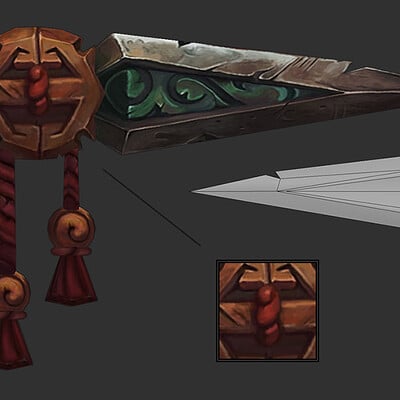The image features a dark gray background with an eclectic assortment of ancient artifacts. Dominating the right-hand side is the tip of a sword, marked by a small niche on the top portion. Just above the sword tip, a mysterious object appears, resembling a part of another sword but encasing an emerald within bronze. This could be an artifact. To the left, a circular wooden face with two braids, held together by shells, adds a tribal, rustic charm. Below, a square wooden face beams with a broad smile, hair cascading over the top corners of its eyes, further enhancing the antique aesthetic. Additionally, a dark green triangular artifact with light gray edging, a silver rectangle with black lines, and a design incorporating dark brown, gold, and red hues adorn the scene. These intricate objects, possibly part of an ancient collection, are connected by ornate, woven ropes, suggesting a deeply historical or ritualistic significance.